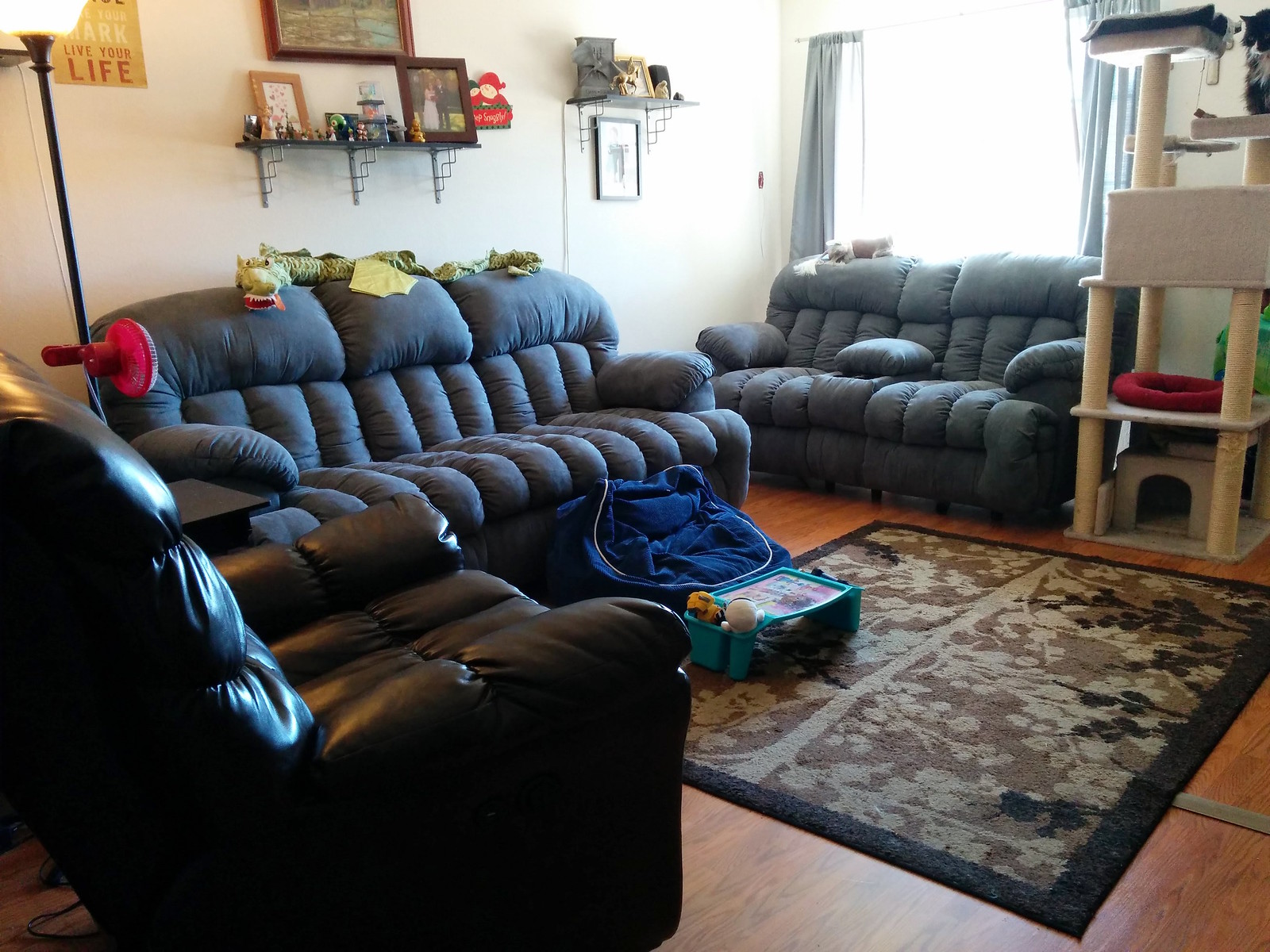This photograph showcases a well-organized living room with white walls and large terracotta-tiled flooring. Central to the room are two plush, puffy-armed couches: one in a darker blue and the other in a lighter blue, almost forming an L-shape. A dark brown leather or vinyl recliner complements the seating arrangement. A large window behind the blue couch, adorned with matching blue-gray curtains, floods the space with natural light. Next to this couch is a tall, tan cat tree, featuring cream-colored carpeting and a small red cat bed on one level. At the top of the tree, nearly out of frame, are two cats, one of which is black and white. The room's focal point is a multi-toned brown and cream rug, with a medium-brown, light-brown, and cream pattern. Scattered around it are children's toys, including a plastic tray with compartments and what appears to be a dark blue bean bag chair. Shelving on the walls holds photographs and various knick-knacks, while a floor lamp with a little red fan attached to its dark stem stands near the couches. Lastly, a long green dragon stuffed animal lies atop the couch against the wall, adding a whimsical touch to this inviting and sunlit living space.